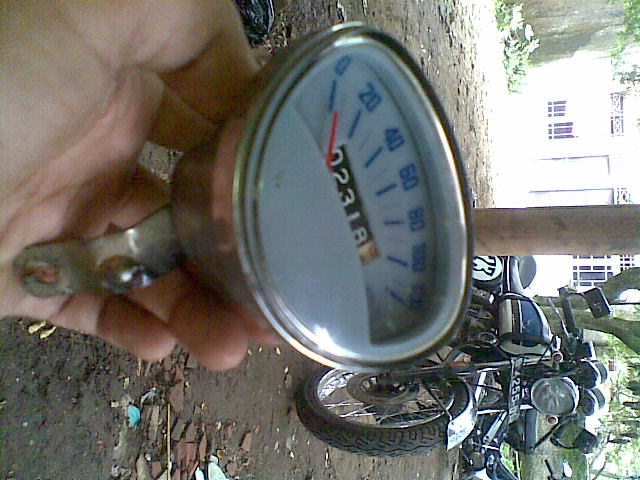This photograph, rotated 90 degrees, features a detailed close-up of a motorcycle's control panel being held by someone's left hand. Central to the image, a blue dial with numbers ranging from 0 to 120, likely representing the speedometer in miles per hour, stands out. Adjacent to it, a recessed panel displays the odometer readings in white numbers on a black background, marking 02318.3 miles. 

In the background, a blue motorcycle bearing the number 23 is visible, casually leaning against a light post, hinting at its everyday use rather than a showpiece. The ground underneath is a mix of compacted shale or dirt, scattered with fragments that might be pottery. Adding to the scene is a weathered and somewhat indistinct building, contributing to a rustic atmosphere. The photograph is taken during the daytime, with natural light providing clarity to the scene. Overall, the image conveys a sense of adventure and wear, capturing the essence of a well-used and cherished motorcycle.